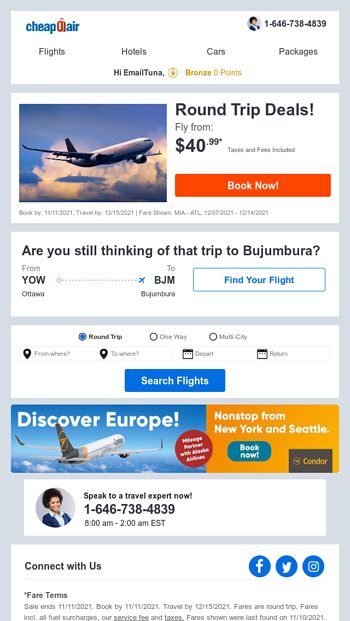The image displayed on the webpage belongs to Cheapo Air, evidenced by the prominent blue and red Cheapo Air logo in the upper left-hand corner. In the upper right, a slightly blurry avatar within a circle is visible, accompanied by the phone number 1-646-738-4839. Below the header, there are navigational options for "Flights," "Hotels," "Cars," and "Packages."

Following this, the user interface greets the visitor with options to interact, labeled "Hi, Email, Tuna, Bronze, and Zero Points." Directly underneath, an image captures a commercial airplane flying through the blue sky, surrounded by white clouds, heading towards the right. Accompanying this image is a bold offer: "Round-trip deals fly from $40.99," marked with an asterisk indicating additional details. An orange call-to-action button labeled "Book Now" appears prominently in white font.

Additional fare details state: "Book by 11-15-2021, Travel by 12-10-2021. Fare shown MIA to ATL (Miami to Atlanta) from 12-07-2021 to 12-14-2021." An adjacent prompt inquires if the user is "still thinking of that trip to Bujumbura?" It specifies the route "YOW (Ottawa) to BJM (Bujumbura)," followed by a clickable "Find Your Flight" link in blue.

Immediately above a blue horizontal search bar labeled "Search Flights" are options for selecting "Round-trip," "One-way," and "Multi-city" travel. These options feature corresponding clickable circles, with "Round-trip" highlighted in blue as the current selection.

Another promotional section below encourages users to "Discover Europe," showcasing another airplane flying to the right against a similar scenic sky but angled away from the viewer. The central red dot with text partially obscured indicates a partnership: "with Alaska Airlines." This offer mentions "nonstop flights from New York and Seattle," urging viewers to "book now on Condor."

This section is followed by the same avatar of a smiling woman with dark hair, identifiable in a white Peter Pan-collared shirt beneath a blue long-sleeve jacket, captioned with "Speak to a travel expert now" and the phone number 1-646-738-4839. Customer service hours are listed as "8 a.m. to 2 a.m. EST."

To engage further, social media icons for Facebook, Twitter, and Instagram are displayed under a "Connect with us" heading. Lastly, fare terms are reiterated: "Sale ends 11-11-2021; book by 11-11-2021; travel by 12-15-2021. Fares are round-trip and include all fuel surcharges, service fees, and taxes." It is noted that these fares were most recently found on 11-10-2021.

This webpage targets users searching for affordable travel options with Cheapo Air.